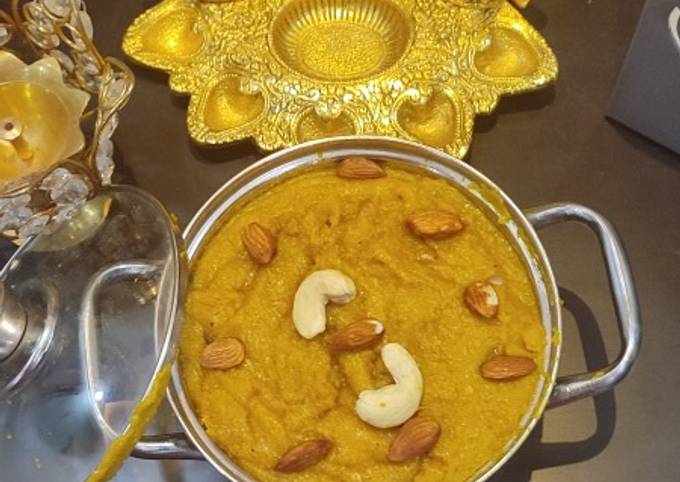The photograph features a large silver pot with two metallic handles, positioned centrally at the bottom of the image, resting on a shiny brown surface. Inside the pot, a golden, pasty halwa is visible, dotted with various nuts including about eight almonds and two cashews. A clear lid with a silver rim leans against the pot on the left side, with a bit of the halwa transferring onto the outside rim. The scene is enriched by an ornate, golden decorative centerpiece located at the top center of the image. This centerpiece has a large central compartment, possibly for chips, and several heart-shaped compartments extending outwards, likely for sauces. Additionally, an item resembling a bejeweled and golden candle holder is visible to the left, and a black box is discernible in the top right corner of the photograph.